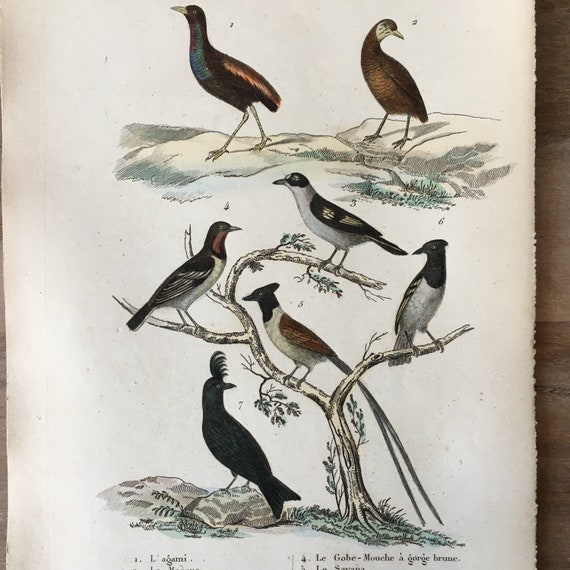The image appears to be a detailed, hand-drawn illustration from an old book, likely created using colored pencils. It is displayed on a thick, older piece of paper set against a brown wooden surface. The illustration is divided into two sections. The top section features a rocky landscape with two long-legged, long-necked birds. The first bird is predominantly black with green and yellow coloring on its neck and wings, and it faces left. The second bird is brown with a yellow beak, a distinctive white face, and is looking backward over its shoulder.

The bottom section showcases a tree with four branches and a bird standing underneath. The tree is populated by four distinct birds. On one branch sits a black-headed bird with a white body. Another bird, with a striking red body, red wings, a white body, and black head, has notably long tail feathers. At the top of the tree is a bird with black around its eyes, a white body, and black and white speckled feathers. The final bird on this branch has a red area under its eye, a black head, and a combination of white and black feathers with a white body. The bird standing under the tree is entirely black.

The illustration exudes a sense of intricate detail and diversity among the birds, each species carefully depicted in varying colors and forms. The overall page is white, containing snippets of text and some numbers partially cut off at the bottom. This meticulously crafted drawing captures the essence and beauty of the birds and their natural surroundings, emphasizing the variety in species and distinctive markings of each bird.